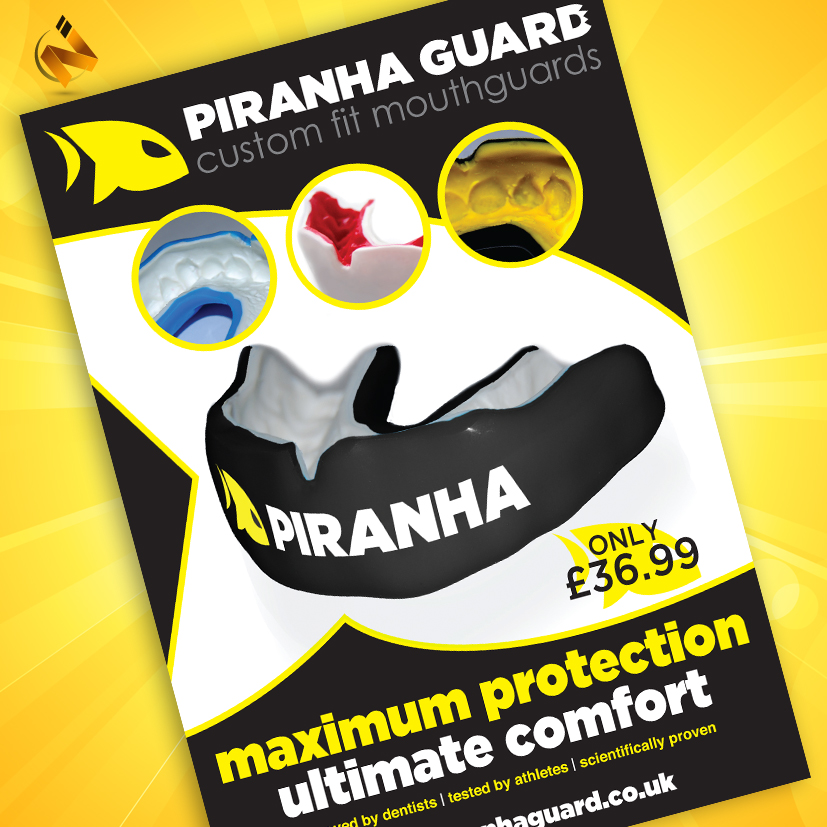This vibrant advertisement for Prana Guard Custom-Fit Mouth Guards boasts a striking design, centered on a yellow sunburst background with radiant beams emanating from the middle. The ad itself is prominently displayed on a leaning rectangle, skewed towards the top left. At the top, bold white text announces "Prana Guard Custom-Fit Mouth Guards," alongside a playful yellow piranha logo.

Below the header, three circular thumbnails showcase different aspects of the mouth guards: the first circle features an image of a mouth guard, the second is unclear but includes red and white elements, and the third displays yellow teeth. Dominating the main segment of the rectangle, a detailed image of the mouth guard highlights the piranha logo and the price, "Only 36.99 Pounds."

The bottom section of the ad emphasizes the product's merits, with phrases like "Maximum Protection, Ultimate Comfort" in visible, albeit partly cut-off, yellow text. Beneath these claims, additional assurances state, "Tested by Athletes, Scientifically Proven," and a small white URL, guard.co.uk, is positioned at the very bottom.